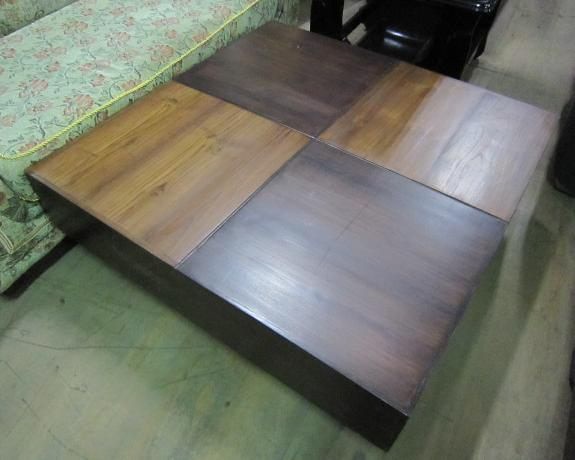In the image, a worn, two-toned wooden coffee table sits prominently in the center. The table, designed in a 2x2 checkerboard grid pattern with alternating squares of light and dark brown wood, shows signs of age with its unvarnished and non-shiny surface. The floor beneath the table is gray, appearing like scuffed hardwood or laminate. Pushed up against the table's left side is a light green couch adorned with a red floral pattern. In the upper right corner, a partial view of a black chair or structure is visible. The scene, captured from a top-down angle under what seems to be fluorescent lighting, suggests an indoor setting, perhaps a furniture store or a living room.